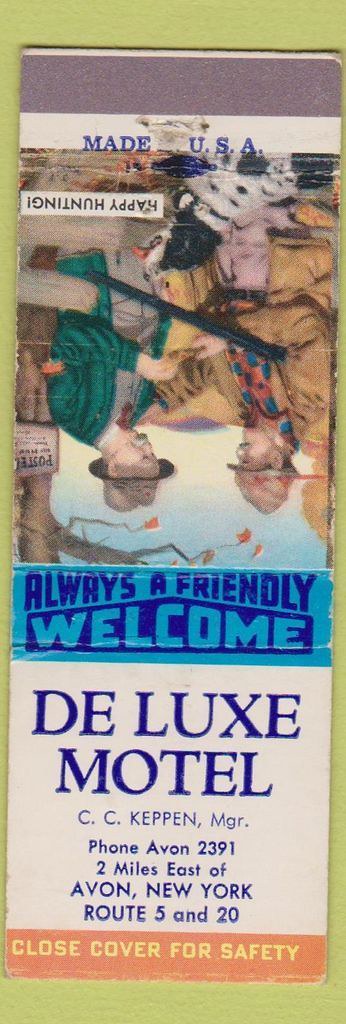The image depicts a fully opened matchbook cover against a light green background. The left side, oriented upside down, features an illustrated scene likely from the 1940s of two Caucasian men with a black and white dog positioned between them. The man on the left wears a long brown jacket and holds a double-barrel shotgun, while the man on the right, donning a green jacket and brown hat, appears to be handing something, possibly a cigar, to the other man. Below this illustration, in blue text, is the phrase "Happy Hunting." 

At the top of the matchbook's inner cover is a light grayish-purple banner followed by a white strip and a blue stamp stating, “Made USA”. Below this illustration, but oriented correctly, is blue text exclaiming "Always a friendly welcome." The lower portion includes a white background with blue print that reads: "Deluxe Motel, C.C. Kepin Manager, Phone Avon 2391, two miles east of Avon, New York, Route 5 and 20.” Finally, an orange footer with yellow text advises, "Close cover for safety."